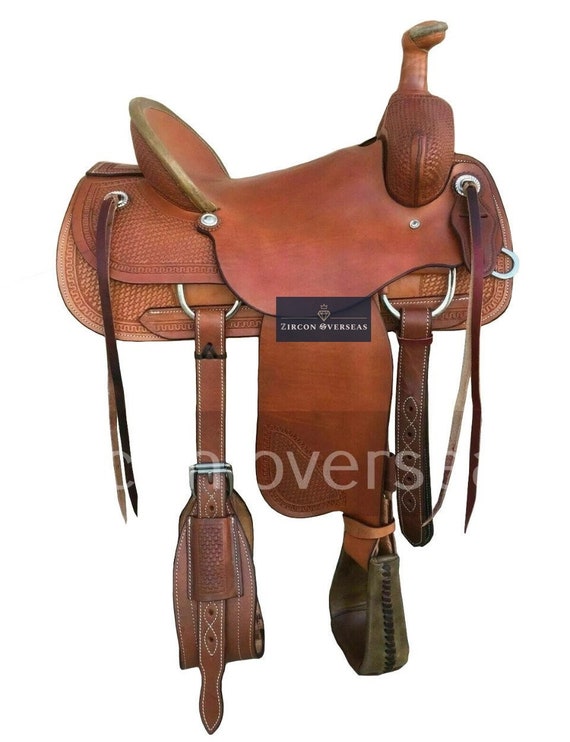The image displays an intricately designed brown leather saddle, featuring meticulously detailed stitching along its seams. Dangling from various parts of the saddle are decorative leather tassels, adding an element of traditional craftsmanship. The saddle includes two sturdy stirrups meant for securing the rider's feet, enhancing comfort and stability. There are two cinch straps designed to firmly fasten the saddle to the horse, ensuring a safe ride. 

Topping the saddle is a prominent horn, commonly used for gripping or tying a rope during riding activities, particularly in ranching or rodeo events. Situated at the rear of the saddle is a short, yet supportive backrest, preventing the rider from sliding backward. Adding a touch of modern branding, the saddle displays a black label printed with "Zircon Overseas" in bold, white lettering. This name is also subtly overlaid on the saddle in a translucent white font. The overall design balances functionality and style, making it a noteworthy piece of equestrian equipment.